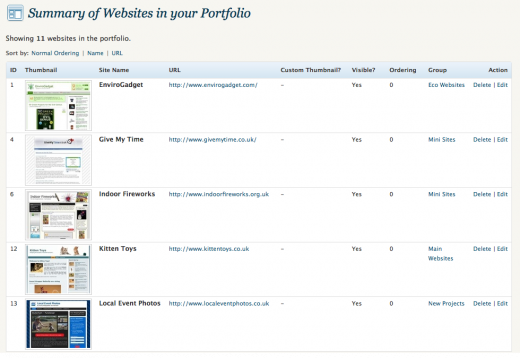Here is a cleaned-up and highly detailed caption for the image:

---

The image is a screenshot from someone's computer, displaying a web management interface. At the very top, there is a gray banner. In the top left corner of this banner, the text "Summary of websites in your portfolio" is written in blue font. Below this, it states, "Showing 11 websites in the portfolio," accompanied by sorting options set to "Normal ordering."

On the left side, there are numbered entries: 1, 4, 6, 12, and 13. Each entry includes a thumbnail image, site name, URL, custom thumbnail, title, visibility status, ordering information, group designation, and action buttons. The entries are as follows:
- Entry #1: Named "EnviroCadet."
- Entry #4: Named "Give My Time."
- Entry #6: Named "Indoor Fireworks."
- Entry #12: Named "Kitten Toys."
- Entry #13: Named "Local Event Photos."

The background of the page is white, with black text. URLs, group names, and action links are highlighted in blue.